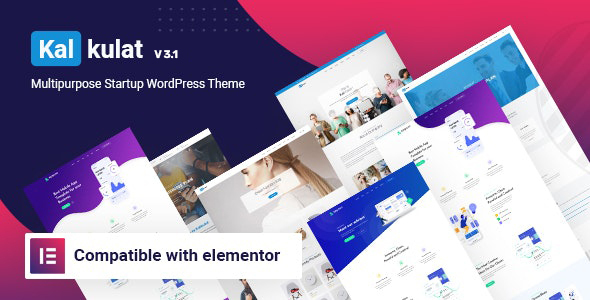This image serves as an advertisement for "Calculot Version 3.1," a versatile startup WordPress theme. The ad highlights its compatibility with Elementor, a popular page builder. It showcases a variety of pre-designed WordPress themes, which appear to be standard templates often selected for business websites. These themes feature typical stock photos, including scenes of people engaged in office settings, animatedly discussing projects, and standing against walls in friendly, inclusive group poses. The individuals shown are of diverse racial backgrounds, reflecting a modern and inclusive workplace. The themes employ common color schemes such as blue-and-white or purple-and-white, lending them a professional yet somewhat predictable appearance. Overall, the ad presents multiple clean yet generic design options available for website customization.